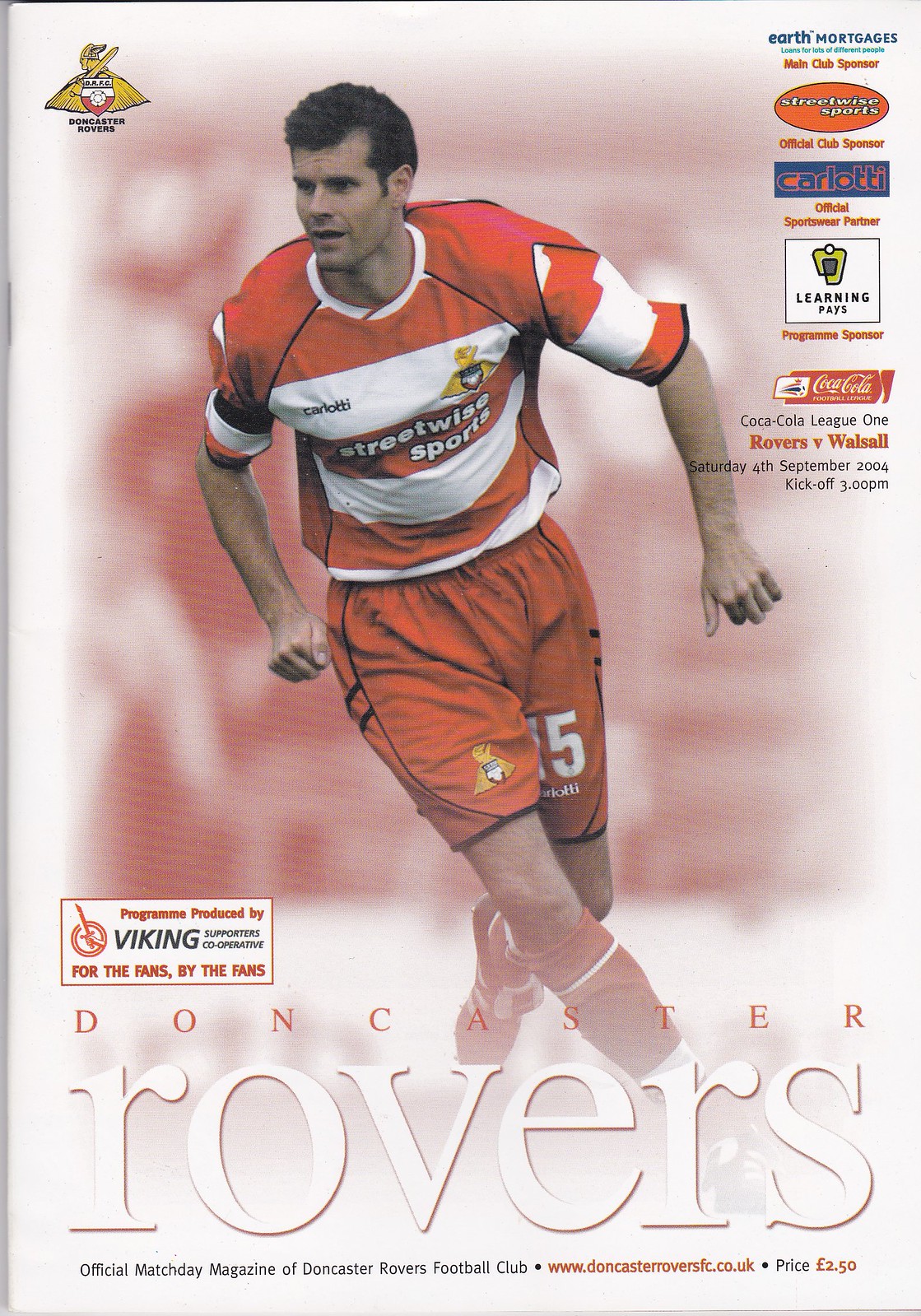The image depicts the front cover of the official match day magazine for Doncaster Rovers Football Club. Centrally featured is a football player in a red uniform with white stripes, red shorts, and a panel across his chest displaying the sponsor "Streetwise Sports." The background is primarily white, with red elements prominently highlighting the magazine's title and other text. In the upper left corner, there's a logo resembling an eagle, while various business logos line the upper right corner. At the bottom, the magazine notes that it is "Program Produced by Viking, Supporters Cooperative, for the fans, by the fans," and identifies itself as the "official match day magazine of Doncaster Rovers Football Club." The price is listed at £2.50, and the website, partially visible, ends with ".co.uk" indicating its British origin. The overall design emphasizes the club’s red and white colors, embedding various details and sponsors into its layout.